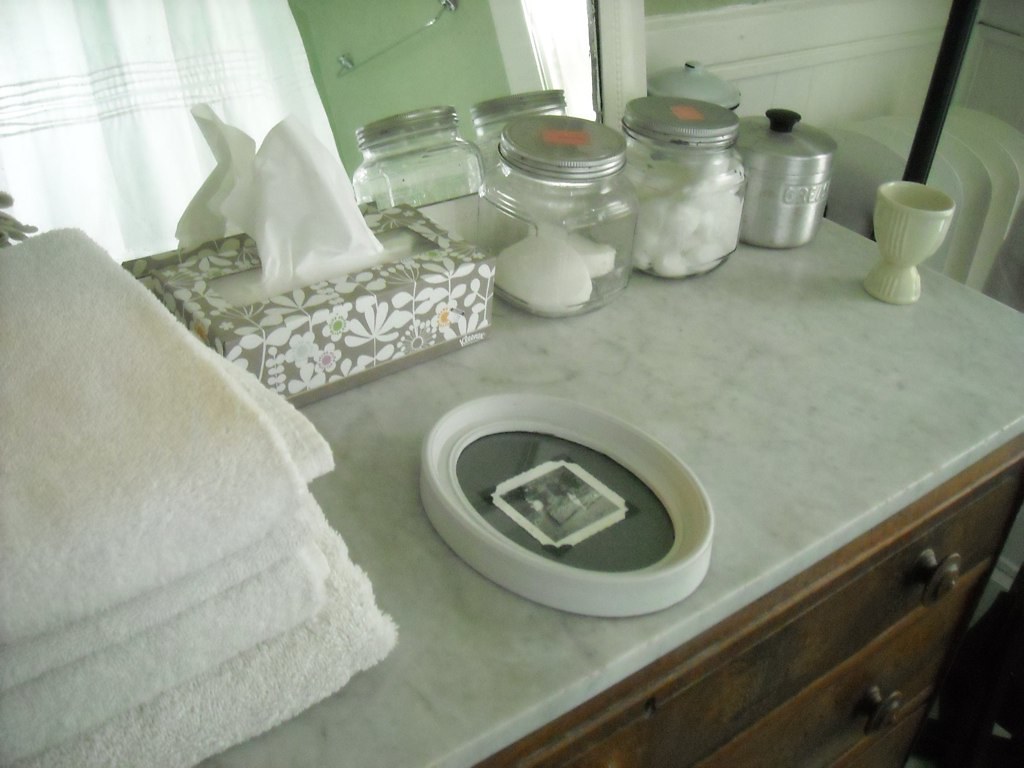The image showcases a section of what appears to be a vintage-styled bedroom, though it could initially be mistaken for a bathroom due to certain elements. The focal point is a dresser with a white stone top. Positioned on the left side of the dresser are neatly folded white towels. Centrally placed is a box of tissues, while to the right, a collection of small glass and silver jars containing items like cotton swabs is meticulously arranged. Centrally on the dresser sits a white and black saucer. No text accompanies the image, allowing the intricate arrangement and decor to speak for themselves. The overall aesthetic of the room, with its carefully placed objects and choice of furniture, exudes an old-timey, vintage charm reminiscent of the 1950s.